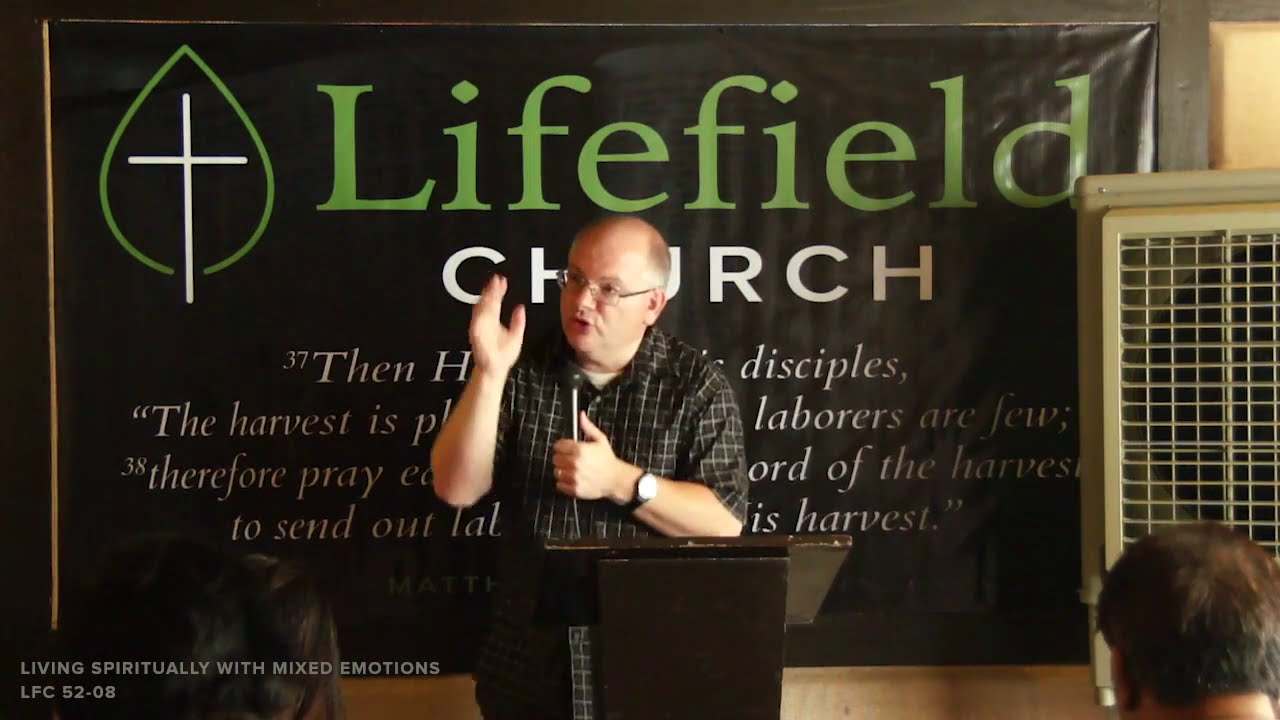In the image, a Caucasian man, likely a pastor, is captured as he preaches at Life Field Church. He's wearing a short-sleeved, black and gold checkered button-down shirt, and he has a watch on his right wrist. The man is bald with glasses and some gray hair on the sides. He is holding a black microphone in his left hand, while his right hand is raised as he speaks passionately to the congregation.

Behind him, a large, black, rectangular banner prominently displays the words "Life Field Church" with "Life Field" in green and "Church" in white. A distinctive logo featuring a green leaf with a white cross through it can be seen on the left of the banner. There is also a white Bible verse quote partially obscured by the pastor. 

To the far left of the image, there is a dark brown wooden podium, and nearby, what appears to be a large white fan or cage is visible. At the bottom left of the image, the phrase "Living Spiritually with Mixed Emotions, OFC 5208" is written, which might indicate the topic of the sermon. In the bottom right, the back of a person's head can be seen, likely someone listening to the sermon. The scene conveys a spiritual and intimate atmosphere within the church setting.